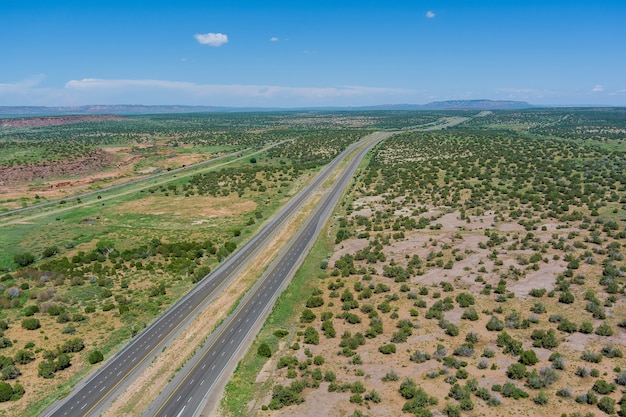An aerial photograph taken during the daytime showcases a long, multi-lane highway extending from the lower left corner of the image and curving slightly towards the upper right. This road stretches endlessly into the flat horizon until it converges with what appears to be a distant mountain range. The landscape is a patchwork of sparse greenery and brown terrain, with grassy areas punctuated by patchy bushes, predominantly in the upper sections, while the lower right corner is more barren. Prominent strips of land flanking the highway have arid stretches and sparse tree cover. The sky is mostly clear with a small puff of cloud just left of the center, two smaller clouds to its right, and a distant line of clouds on the left. The vibrant blue skies and the sun create a stark contrast with the earth-toned landscape below.